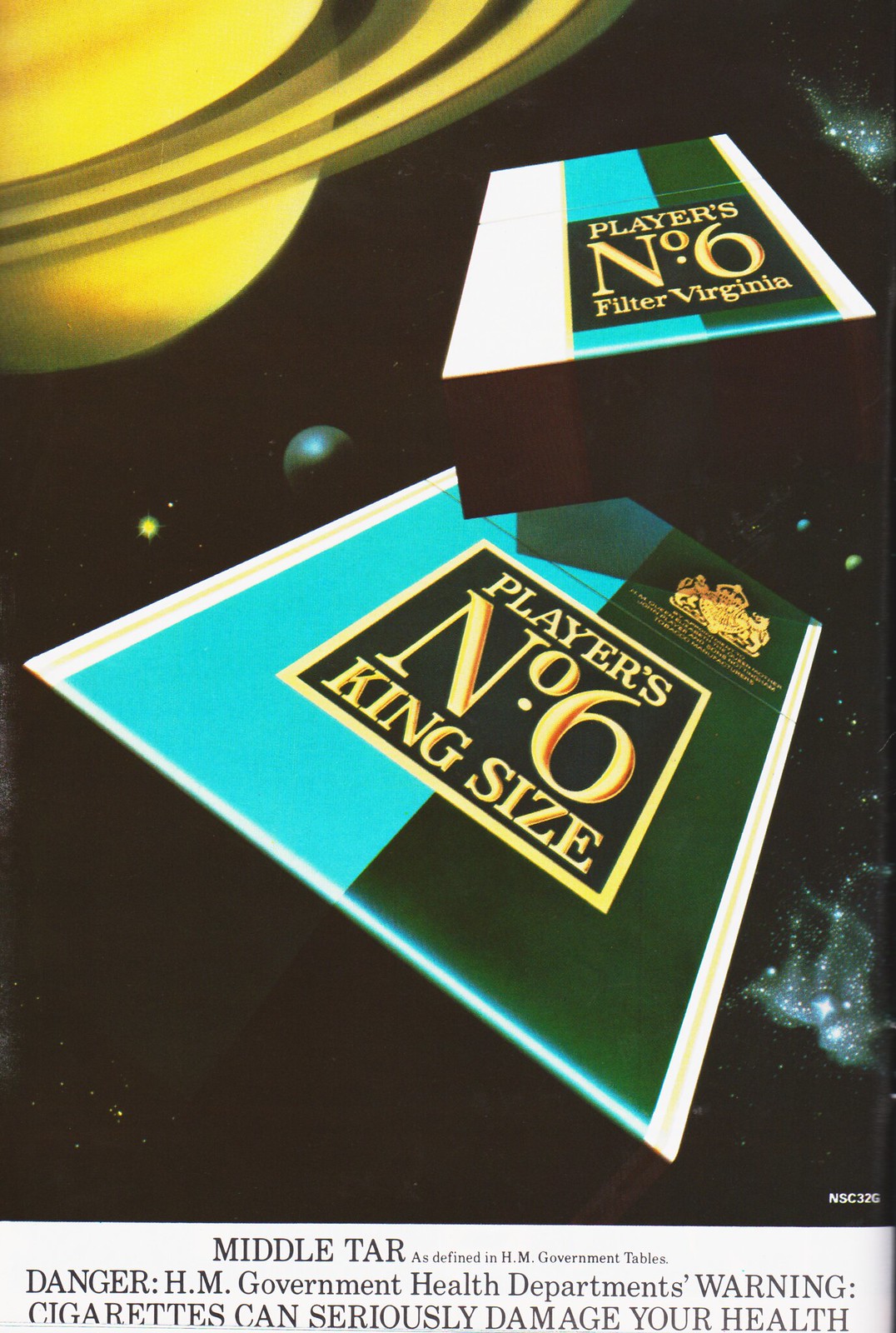The promotional flyer features two cigarette boxes prominently displayed against a black background adorned with realistic, stylized space-themed artwork, including stars and various planets. At the top center of the image, a large yellow planet with a dark grey and yellow rim, resembling Saturn, dominates the scene. Two more smaller planets and a bright yellow star are dispersed across the middle and right side of the background.

In the central portion of the image, the two cigarette packs appear to be floating in space, positioned to create a sense of depth. The closer pack is larger, while the farther one is smaller. Each box features a light blue side and a dark green side, along with a yellow square containing multiple lines of yellow text. The text on the cigarette packs reads, "Players, Number Six, Filter, Virginia," and "King Size." A black stripe at the bottom of the flyer bears the warning: "Middle Tar, as defined in HM Government tables. Danger: HM Government Health Department's warning: Cigarettes can seriously damage your health," with the code "NSC-32G" appearing in the bottom right corner.